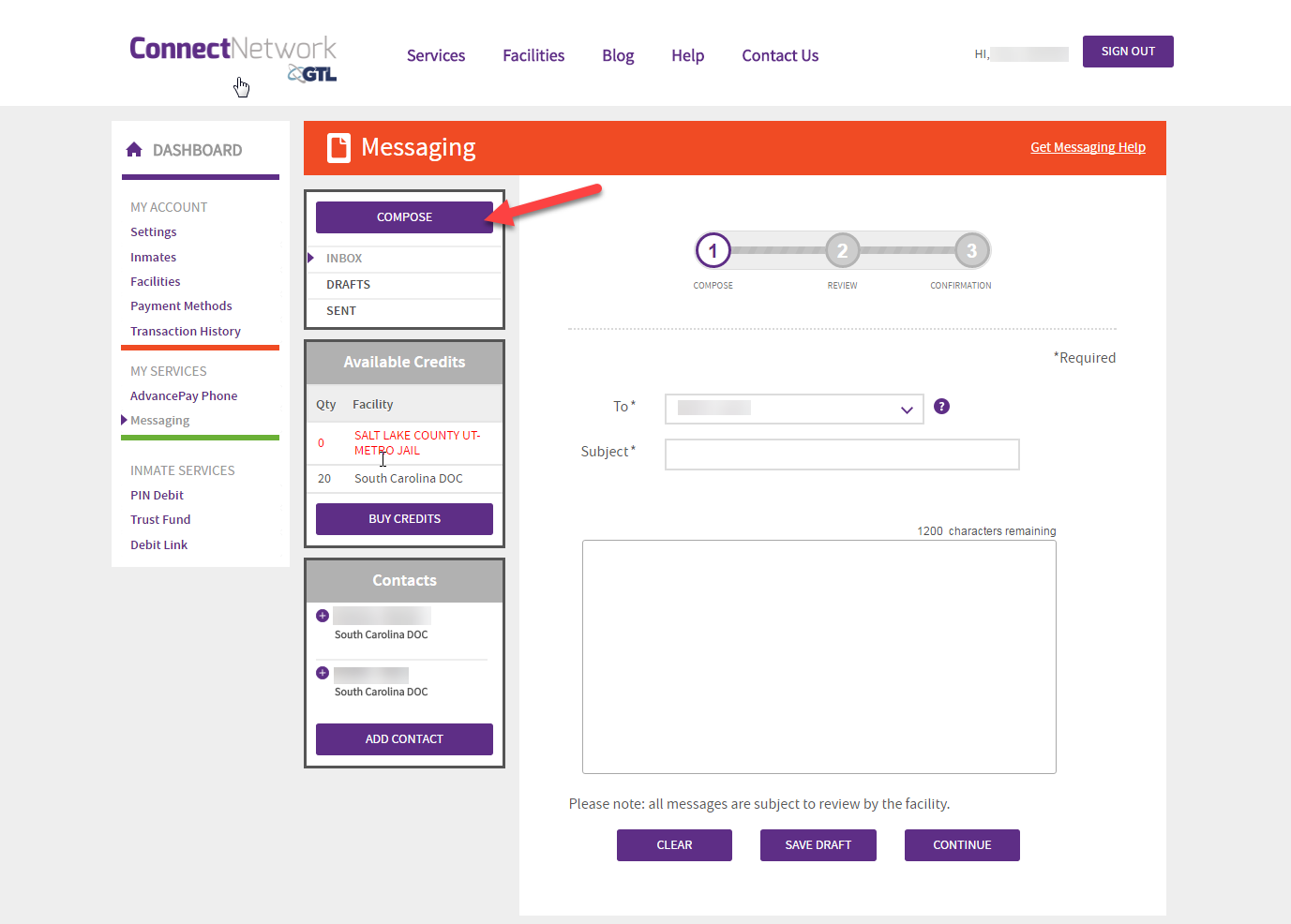The image features a detailed screenshot of a business application interface, specifically tailored for managing inmate communication and services. In the top left corner, the application is branded "Connect Network" with an adjacent GTL icon. Directly to the right, a navigation menu displays in purple text against a white background, listing Services, Facilities, Blog, Help, Contact Us, and Sign Out. A blurred name shows at the top right, indicating a logged-in user.

Below the Connect Network header is a prominent dashboard labeled "DASHBOARD" in all capital letters, complemented by a home icon. The screen’s primary color scheme is white, with highlights in purple. Dominating the screen is a striking orange banner that indicates the user is currently in the "Messaging" section.

On the left sidebar, various sections are listed: My Account, Settings, Inmates, Facilities, Payment Methods, and Transaction History. Under these main sections, there's a "My Services" tab featuring Advanced Pay Phone. Below that, Messaging and Inmate Services options include PIN Debit, Trust Fund, and Debit Link.

In the center of the screen is a prominent purple "Compose" button, accompanied by an orange arrow pointing to it. Below this button, tabs for Inbox, Drafts, and Sent are visible. Further down, an Available Credits box and a Contacts box provide additional user information and options.

The focal point of the image is a large form in the center designed for composing an email or message. This form includes a sizeable text box for the email content, a Subject box, and a "To" dropdown for selecting the recipient. At the bottom of the form are three purple buttons labeled "Continue," "Save Draft," and "Clear," streamlining user actions within the application.